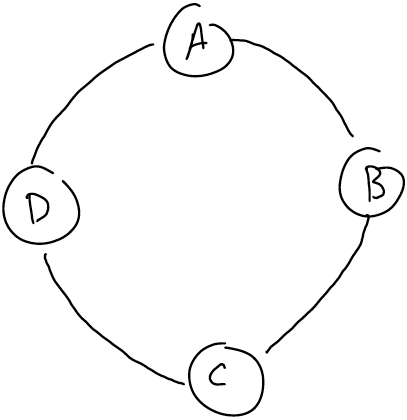This pencil-drawn image features a large circle with four smaller circles positioned along its perimeter, representing a roughly compass-like arrangement. The smaller circles are situated at the top, right, bottom, and left of the main circle, encasing the letters A, B, C, and D, respectively. Despite the slight misalignment of the smaller circles, the overall design clearly indicates a clockwise progression from A at the top, B on the right, C at the bottom, and D on the left. The letters, written in uppercase, are easily legible despite the uneven handwriting. This straightforward and simple line drawing effectively conveys a methodical arrangement of labeled points within a circular frame.